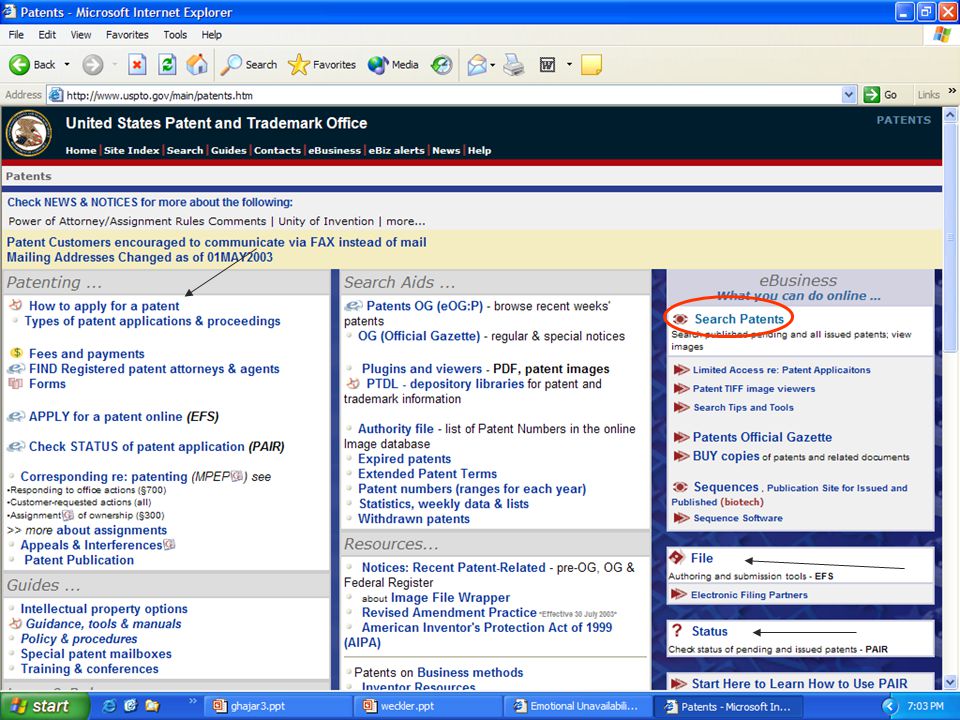The image is a detailed screenshot from a laptop displaying a webpage in landscape mode, specifically from the United States Patent and Trademark Office (USPTO) website. The upper left-hand corner indicates that the browser used is Microsoft Internet Explorer, showing 'patents' in light blue text. On the upper right-hand corner, there's an option to close the window.

The page navigation includes standard browser tabs like File, Edit, View, Favorites, Tools, and Help. Below these tabs, there are options to go Back or Forward, and buttons for Search, Favorites, and Media. The address bar displays the URL: "USPTO.gov/Patents.HTM."

The main content frame shows the title "United States Patent and Trademark Office" on a black background. Below this, there's a navigation menu with tabs labeled Home, Site Index, Search, Guides, Contacts, E-business, Ebiz alerts, News, and Help. On the upper right-hand corner of this row, 'patents' is again highlighted.

The main informational area starts with a light blue stripe that reads: "Check news and notices for more about the following: power of attorney, assignment rule comments, unity of invention, and more." It is followed by a section with a yellow background, informing patent customers to communicate via fax instead of mail, noting that the mailing address changed as of May 1st, 2003. A black arrow points to an important message: "How to apply for a patent."

The main body is divided into three columns: the first column is titled "Patenting," the second column starts with "Search," and the third column begins with "E-Business: What You Can Do Online." Drawing particular attention, a big red circle is marked around "Search Patents," indicating the focus of the instructional content.

Further highlighting critical navigation, there are two additional black arrows: one pointing to 'File' and another to 'Status' under relevant sections, elaborating the user's journey to understand how to apply for a patent.